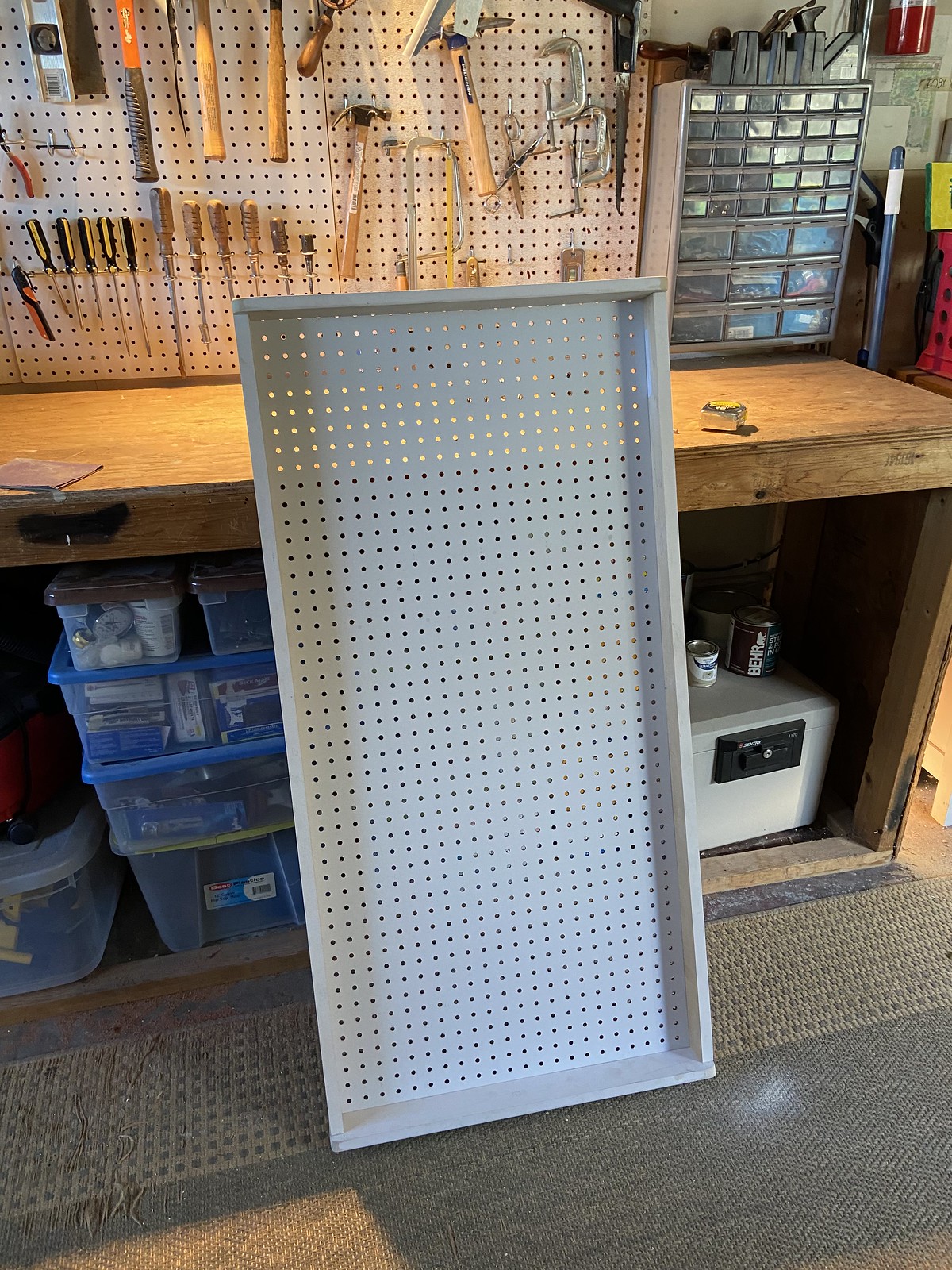The photograph captures a meticulously organized workshop or tool shed. The centerpiece is a long, gray metal tray, approximately three feet high, leaning against a light brown wooden workbench. The tray's surface features a grid of small, circular cutouts. The workbench has a drawer with a handle and is topped with a cork board displaying various tools like screwdrivers, hammers, and a saw, all arranged neatly in rows. To the right, a small cabinet with clear plastic drawers holds various small items, possibly nails and screws. Beneath the workbench, there are clear storage containers stacked on top of each other. The floor is gray with a tan rectangular rug featuring a geometric design. The right side of the image also shows a white object with a few items placed on top of it, possibly a safe, adding to the detailed utility of the space.